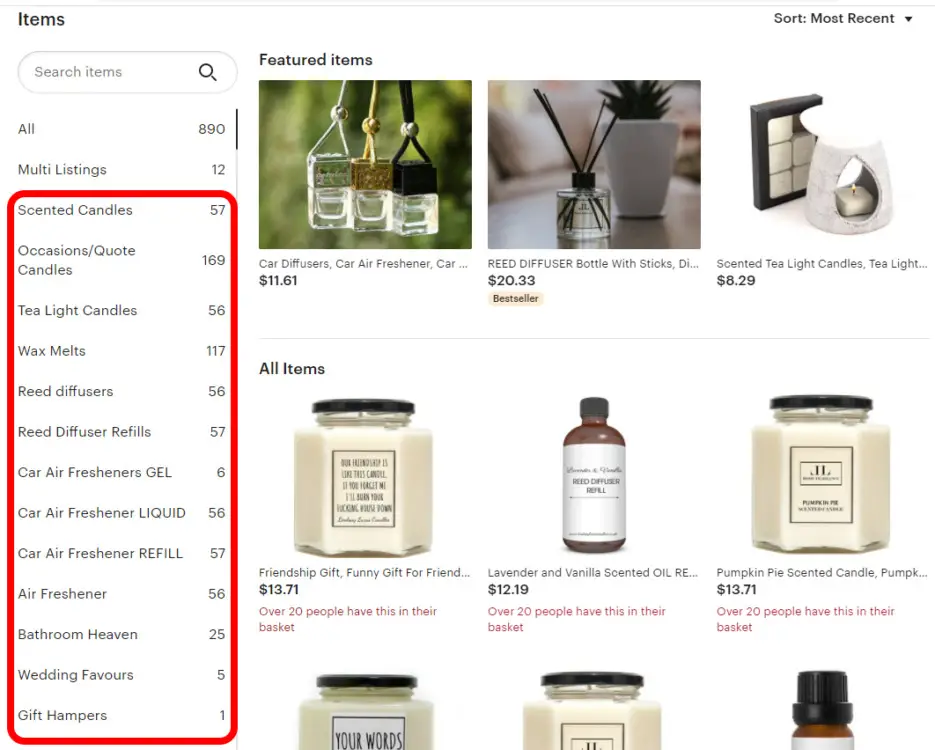This detailed image captures an e-commerce website layout showcasing various products for sale. In the top left corner, the word "Items" is displayed in black text, while the top right corner features a sorting option currently set to "Most Recent." Along the left-hand side of the page, categories are listed with the top two being "All" (890 items) and "Multi Listings" (12 items). Above the categories is a search bar for easy navigation.

Highlighted in a vertical red rectangle are 13 product categories, listed in the following order: 
1. Scented Candles
2. Occasions
3. Quote Candles
4. Tea Light Candles
5. Wax Melts
6. Reed Diffusers
7. Reed Diffuser Refills
8. Car Air Fresheners
9. Gel Car Air Freshener
10. Liquid Car Air Freshener
11. Car Air Freshener Refill
12. Air Freshener
13. Bathroom Heaven
14. Wedding Favors
15. Gift Hampers

Each category displays a number indicating the quantity of items available.

To the right majority of the website, there are three horizontal rows of products. The top row is labeled "Featured Items," displaying products such as car diffusers, reed diffusers, and scented tea light candles, with prices listed below each item. The middle section, marked "Bestseller," highlights a variety of items including a friendship gift candle and a lavender and vanilla scented oil, with another candle positioned on the right. The bottom row features two candles on the left and what appears to be essential oils on the right.

Overall, the layout is thoughtfully organized, providing users with an easy-to-navigate interface to explore a wide range of fragrant products.